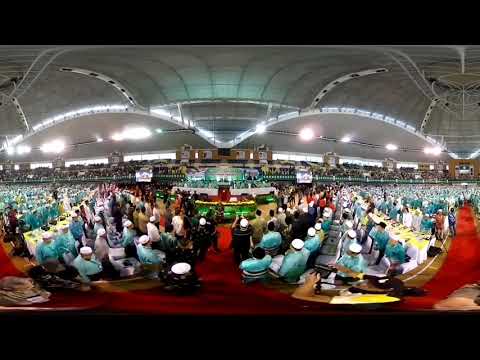In the image, a vibrant crowd of hundreds of people, mostly dressed in light blue shirts and white hats, gathers around a long, rectangular table adorned with a white tablecloth. The crowd sits on a strikingly bright red carpet, which stretches through various aisles within the venue. At the center of attention is a brown podium with individuals standing and presumably speaking to the audience. The setting is grand, dominated by a large, silvery dome ceiling punctuated with numerous lights. This impressive ceiling features two prominent arches creating a rhythmic pattern which frames the scene. The table's centerpieces add splashes of green, brown, and white, contributing to the image's colorful ambiance.